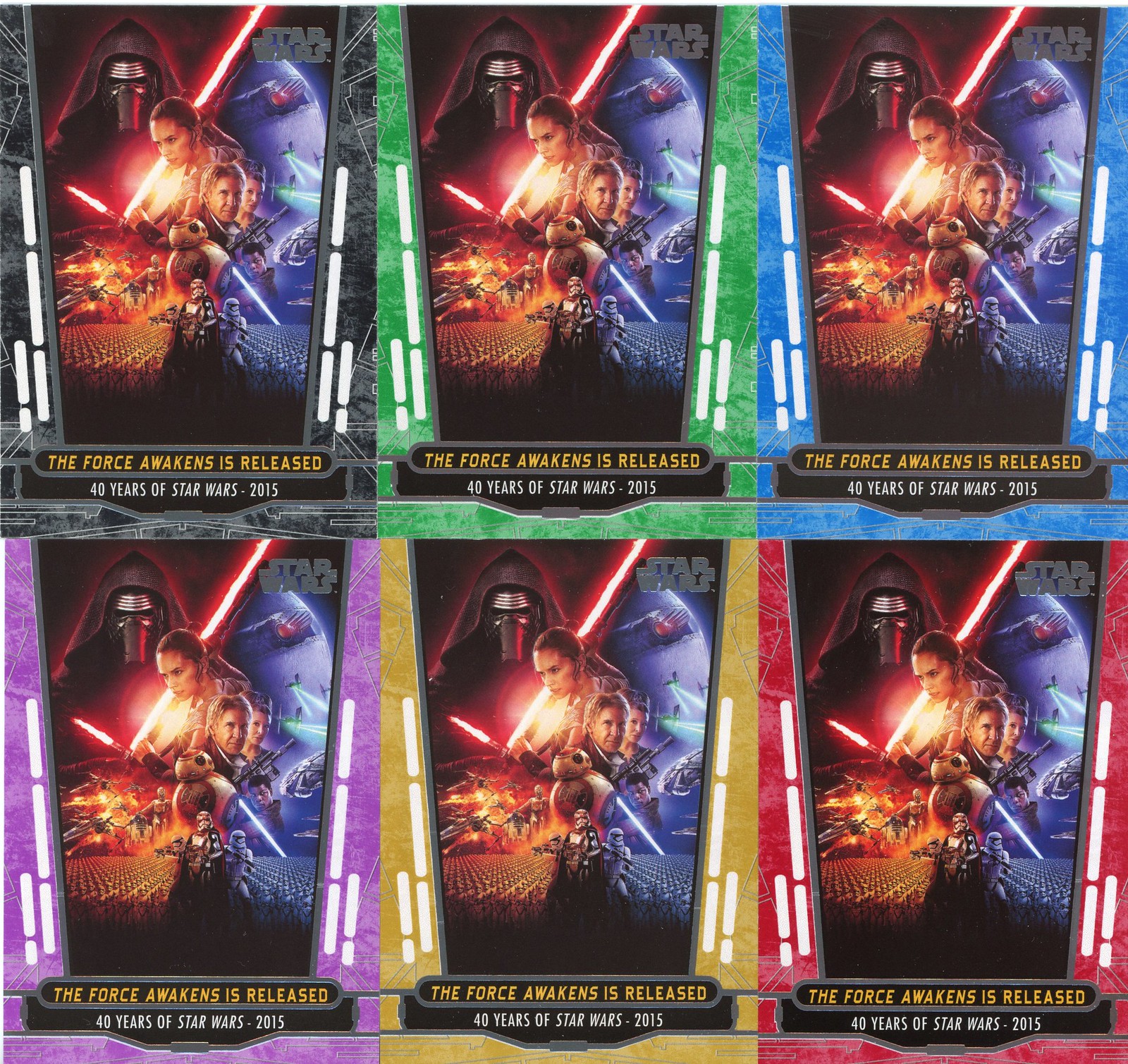The image depicts a series of six versions of the Star Wars: The Force Awakens poster, arranged in a grid with three on the top row and three on the bottom row. Each poster features the same dramatic artwork, showing the main character Rey in an action pose at the center, with the masked antagonist Kylo Ren wielding a red lightsaber behind her, along with appearances of iconic characters like Han Solo and Princess Leia. The poster is dynamically split into red and blue hues, depicting space battles and stormtroopers. These variants appear to be collectible trading cards, likely offered as promotional items when the movie was released. Each card is bordered in a different color—top row from left to right: black, green, and blue; bottom row from left to right: purple, gold/yellow, and red. The text on the cards reads "The Force Awakens is released" in yellow, followed by "40 years of Star Wars - 2015" in white. The upper right corner of each poster features the Star Wars logo in gray.